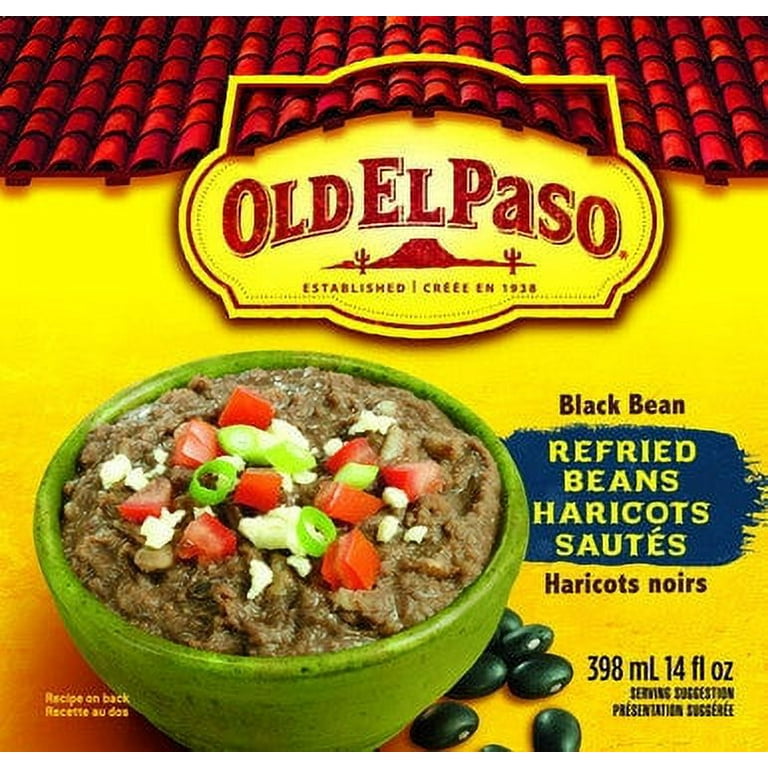The image depicts a box of Old El Paso refried black beans. The box features a distinctive yellow background with a red roof edge, characteristic of Old El Paso’s branding, and the logo prominently displayed. The logo includes the text "Old El Paso, Established 1938," with a stylized shadow effect beneath it. The front of the package also has a large raised mesa graphic between two shadowed cat eyes.

At the bottom left of the box, there is a vibrant image of refried black beans served in a green bowl, garnished with chopped tomatoes, cheese, and green onions. To the right of the bowl, the text on the packaging lists the contents as "Black Bean, Refried Beans, Haricots Salutes." Additional details, like the net contents of "398 milliliters (14 ounces)," are shown on the front. The overall color scheme includes dominant yellows and reds, with accents of brown, white, green, and blue.